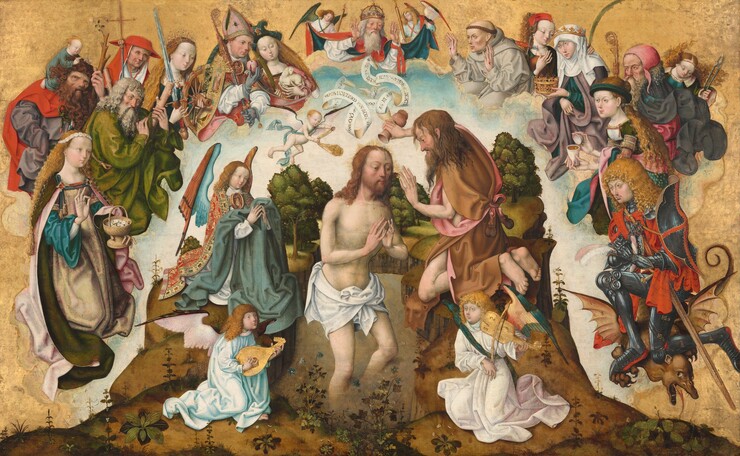The painting is an intricate classical piece, likely from the old world or medieval period. It portrays a significant religious scene, centered on the baptism of Jesus. In the middle of the composition is Jesus, characterized by his fair skin, long brown hair, a mustache, and a beard. He wears only a white cloth around his waist and stands in what appears to be water with his hands partially raised, poised for a prayerful gesture. To his right, a man in brown and tan robes, likely John the Baptist, kneels on a small hill, pouring water from a pot onto Jesus' head and extending his other hand in a gesture of blessing.

Surrounding this central scene, a vibrant atmosphere unfolds with various figures and elements. Below, there's an assembly of winged angels engaged in playing musical instruments—one strums a guitar while another plays a violin or fiddle. Above, cherubic angels, resembling cupids, flutter with white ribbons. To the far right, a knight stands heroically on a demon, brandishing a sword, indicative of a battle between good and evil.

Additional biblical or historical figures populate the background, including women, kings, bishops, and followers, all set against a tan backdrop adorned with towering plants. The elaborate detailing and the array of characters suggest this painting might belong to the 10th century or a similar period.